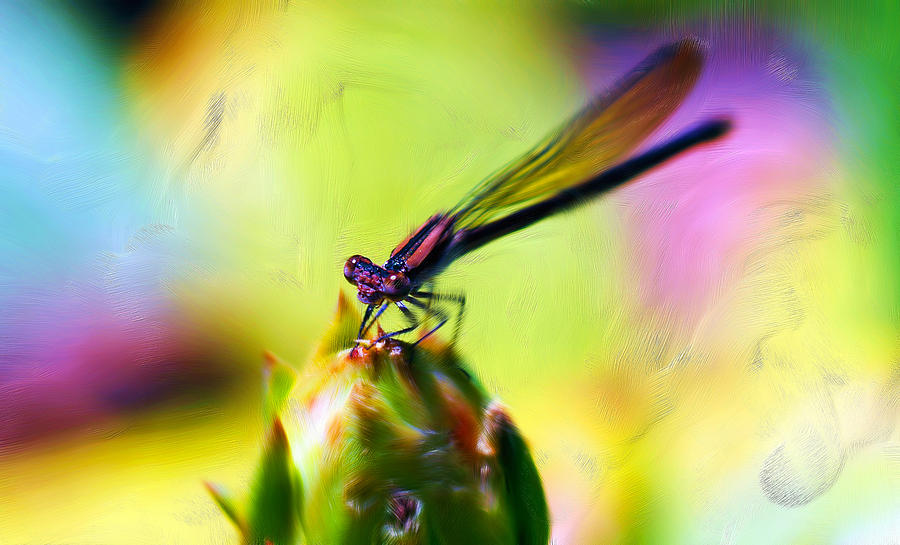The image is an artistic and vibrant representation of a dragonfly perched on what appears to be a flower bud that has yet to bloom. The background, rendered in a spectrum of blurred colors including blue, yellow, green, and purple, evokes the feel of a watercolor painting or a creation generated by an AI model. This blurred background contrasts with the detailed foreground, drawing focus to the main subjects. 

In the foreground, the dragonfly is positioned gracefully in the center of the plant, which resembles a cactus or bud with two rows of dull spikes, tipped with red, on either end. The dragonfly itself features large, bulbous eyes on either side of its head and a long, spindly body. Its wings, described as long and goldish-green, add an additional layer of detail and vibrancy. The dragonfly’s coloring includes shades of dark purple and black, complementing the multi-hued background. This intricate scene captures a moment of natural beauty and tranquility, showcasing the delicate balance of nature.